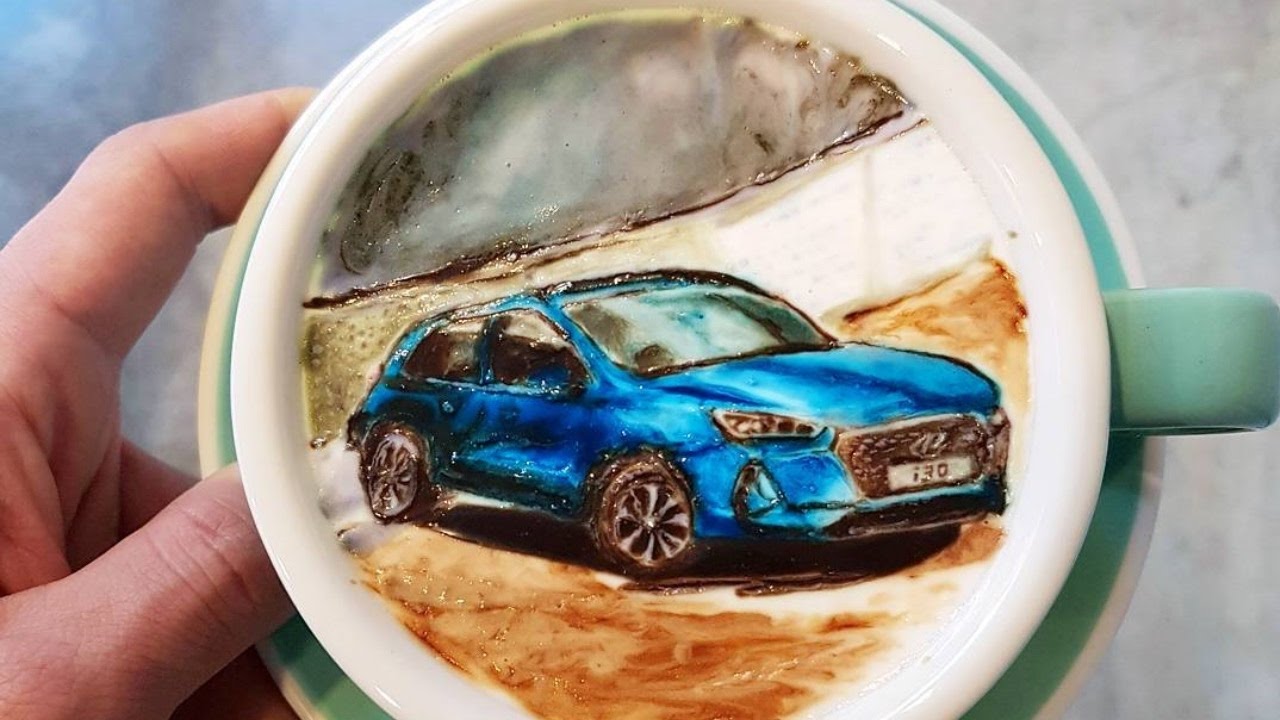This full-color, horizontally rectangular photograph, taken indoors with artistic intent, features a whitish table surface as its backdrop. Dominating the center of the image is a teal-colored coffee cup and saucer set; the saucer has a white border that transitions into a light aqua-green center. The cup, also teal with a white interior, houses a detailed latte art depiction of a blue Hyundai car, complete with the Hyundai emblem and the number "130" on the license plate. This creative foam artwork is surrounded by brown and white hues, adding depth to the design. On the left side of the image, a partial view of a Caucasian hand is visible, showing the palm, thumb, and pointer finger as they hold the saucer. Note the artistic prowess involved in crafting this latte art, making the image both visually captivating and a testament to skilled coffee craftsmanship.